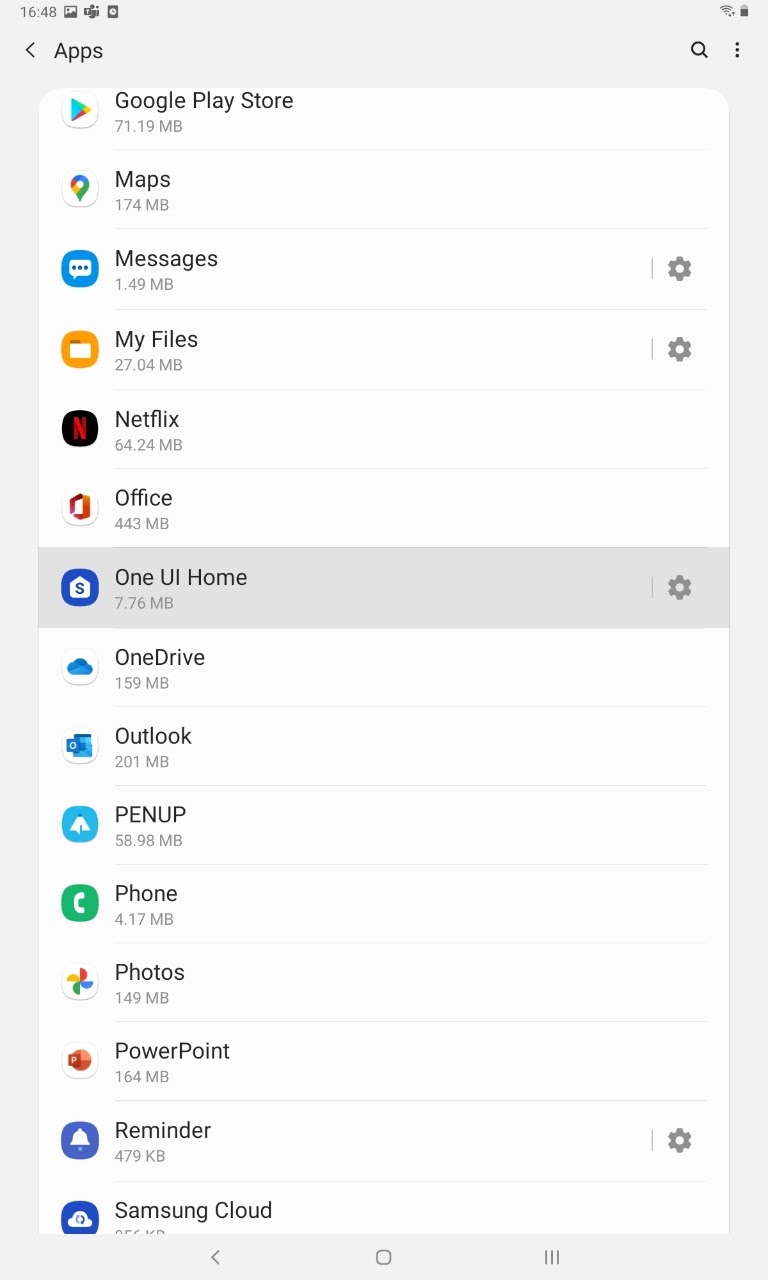Here's a polished and detailed caption for the image described:

"This image is a smartphone screenshot with a white background and a very light gray top border. At the top left corner, the time is displayed in black font as '16:48,' indicating the 24-hour clock format. The screen shows the 'Apps' page, as indicated by the label 'Apps' at the top left. To the right of 'Apps,' there are icons for search and additional options represented by three vertical dots.

The main part of the screen showcases a list of installed apps, each accompanied by its respective logo to the left. The apps listed from top to bottom are: Google Play Store, Maps, Messages, My Files, Netflix, Office, One UI Home (displayed in gray), OneDrive, Outlook, Pen Up, Photo, Phone, PowerPoint, Reminder, and Samsung Cloud.

At the bottom of the screen, the border returns to the same light gray color as the top. In the center of this bottom border is a gray outline of a box, and to the right are three vertical gray lines. An arrow pointing to the left is positioned on the left side of the bottom border."